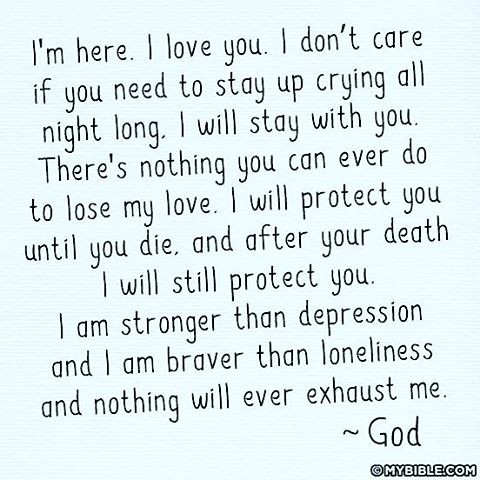The image displays a heartfelt message on a light blue notepad with black lettering. The text reads: "I'm here. I love you. I don't care if you need to stay up crying all night long. I will stay with you. There's nothing you can ever do to lose my love. I will protect you until you die, and after your death, I will still protect you. I am stronger than depression, and I am braver than loneliness, and nothing will ever exhaust me." At the bottom right of the note, it is signed "God," followed by the website "mybible.com." This message, designed to offer comfort and reassurance, serves as a reminder of unwavering divine love and support, particularly for those struggling with severe depression and loneliness.